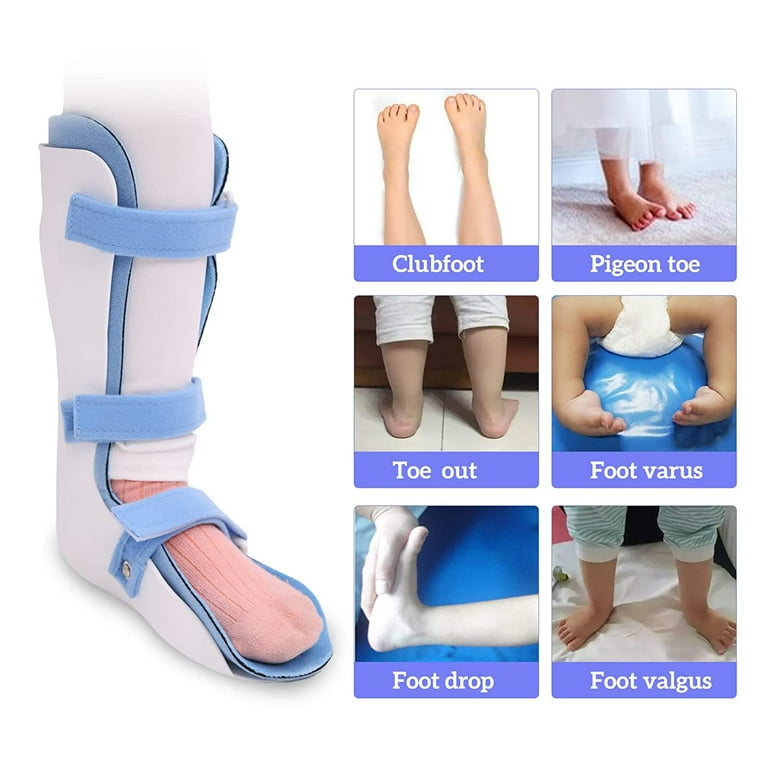The left side of the image displays a left foot encased in a white and light blue aircast or walking boot. The boot features three light blue velcro straps: one across the top of the foot, one at the ankle, and another around the mid-shin. Inside the boot, the foot is clad in a thick pink sock and white leggings that extend up the leg. 

Adjacent to this, on the right side of the image, are six smaller square images arranged in two columns and three rows. Each square showcases a different foot condition with a descriptive label at the bottom against a blue background. 

In the top left square, the condition "clubfoot" is depicted with an image of two bare, misshapen children's feet. The top right square displays "pigeon toe," showing feet positioned inward on a carpet. The middle left square, labeled "toe out," features a rear view of feet pointing outward on the floor. Next, the middle right square labeled "foot varus" shows a baby seated in diapers with curved feet. The bottom left square illustrates "foot drop" with a foot held by a hand, the foot's heel on the bottom and the toes raised. Finally, the bottom right square exhibits "foot valgus," showing feet turned outward, with the child standing on a soft surface like a pillow or mattress.